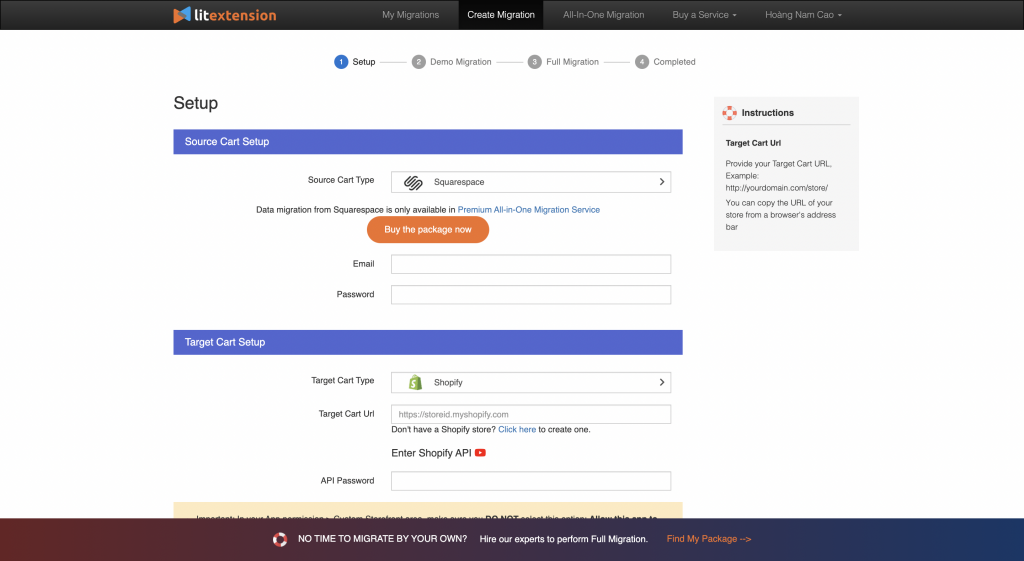This is a screenshot from the Light Extension web page, specifically cropped to exclude web browser information. Light Extension is an online service catering to the migration of e-commerce websites or shopping cart setups. The screenshot depicts the "Create Migration" page, which is currently selected in the dark grey navigational menu at the top. 

The page outlines a structured, four-step migration setup process. It features form fields where users can input details about their source cart, including the cart type, email address, and password required for the migration. Additional fields are provided for the target cart setup, necessitating the correct API information to facilitate the migration. The overall design focuses on guiding users through a detailed and secure e-commerce migration process.